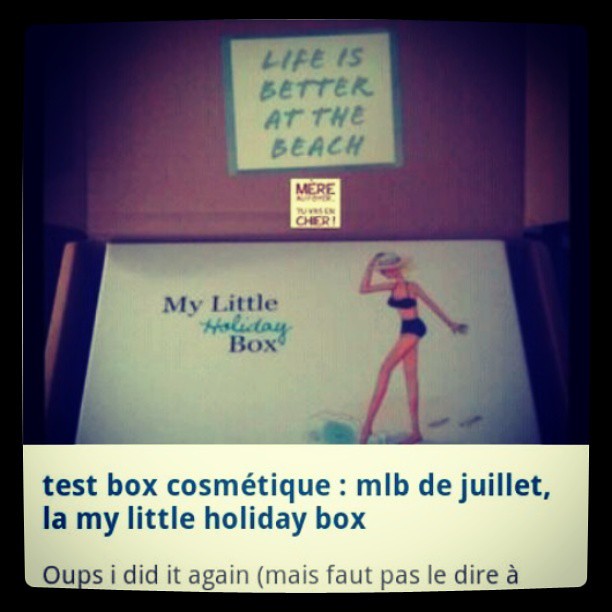The image features a thin black border and a white rectangular box that takes up about a third of the bottom portion of the picture. This white box contains blue text that reads, "Test Box Cosmetique MLB de Joulette La My Little Holiday Box," followed by the phrase, "Oops I did it again." Below this, there's a French phrase: "Mais faut pas le dire," accented appropriately.

The background of the upper part of the image appears purple or possibly brown with a purplish hue. There is an open box here, and on the inside lid of this box, there is a tilted white piece of paper with a blue border, bearing the text, "Life is Better at the Beach," all in capital letters. 

Inside the box is a cartoon drawing of a woman in a bikini, facing left. She is wearing a hat and seems to be stepping onto the sand, indicated by little footprints. Above this illustration, the text reads "My Little Holiday Box," with "holiday" written in cursive.